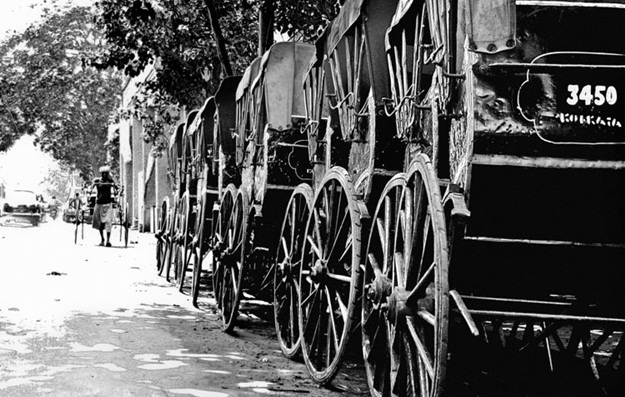This detailed black and white photograph captures a row of rickshaws and carriages lined up along the right side of a tree-lined street. At least five or six of these vehicles are visible, all similar in size with large wheels and black bodies, some featuring canvas roofs and backs. The most prominent rickshaw displays the number "3450" on its back, followed by some illegible letters. In the middle distance, a shirtless man wearing long pants and a hat, likely Indian, seems to be pushing or pulling a rickshaw. The scene suggests the setting might be in India. Additionally, there's more modern traffic in the background, including a motorcycle and a truck, hinting at a blend of traditional and contemporary elements within the same environment. Farther down the street are a few buildings, contributing to the urban landscape captured in this evocative image.